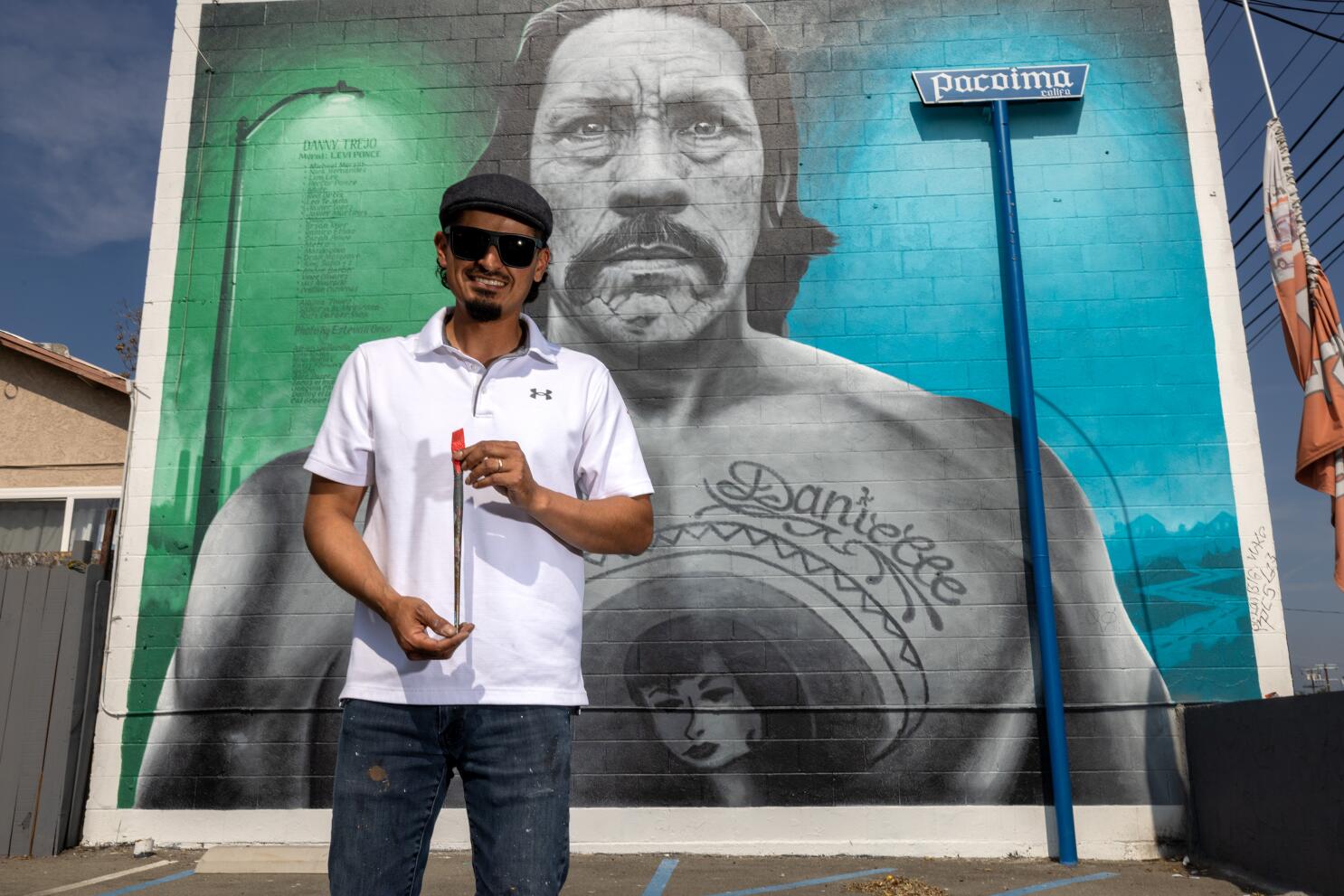The image features a man standing slightly left of center on a sidewalk in front of a large mural. He wears a white short-sleeved polo shirt with an emblem on the left chest, blue jeans, a thin black hat, and dark sunglasses. He has a small goatee and mustache. The man holds a cylindrical object, red-tipped at the top, which tapers to a point, gripping it near his waist with his right hand and higher up with his left.

Behind him, the mural depicts actor Danny Trejo in black and white. Trejo is shirtless, showing a tattoo on his chest that possibly reads "Danielle." He has a thick mustache and long black hair swept back. The mural background is split; the left side features a green backdrop and a painted streetlight with black writing beneath it, while the right side has a blue background. A blue pole with some white writing leans against the wall on the right side of the mural, reaching up to Trejo's forehead level. The word "Pacoima" is visible on the mural. The scene features a clear blue sky in the upper left and a building with a gray fence to the left center, indicating an outdoor setting. The ground is gray asphalt.